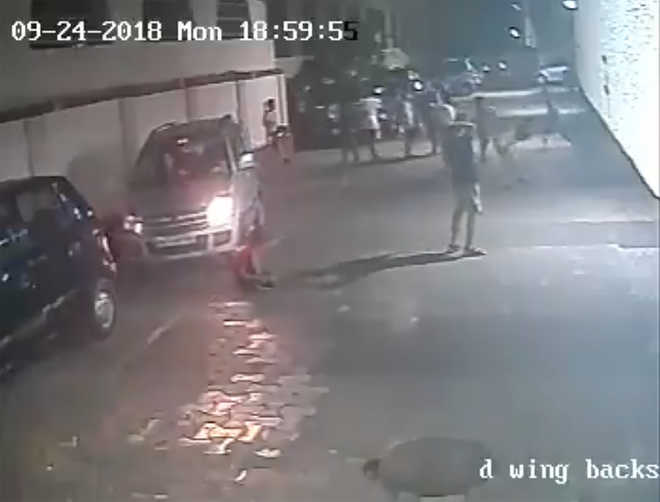The grainy, blurry image appears to be taken at night and shows an outdoor scene, possibly in an alley or a parking lot. The timestamp in white text at the top left corner reads "09-24-2018, Monday, 18:59:55," and the bottom right corner displays "D-Wing backs." The picture is dominated by a cloudy or foggy ambiance, making details hard to discern. Several vehicles line the left side of the image, with a few prominently in the foreground, one of which has its headlights on, though one light might be out. People are scattered around the scene; some stand while one individual appears to be sitting on the ground near the vehicle with the headlight on. The street might be wet, as suggested by possible reflections. Both left and right edges of the photo feature white buildings, adding structure to the scene. Despite the poor image quality, it appears there is some activity, perhaps conflict or observation, as the people and their actions are indistinct.